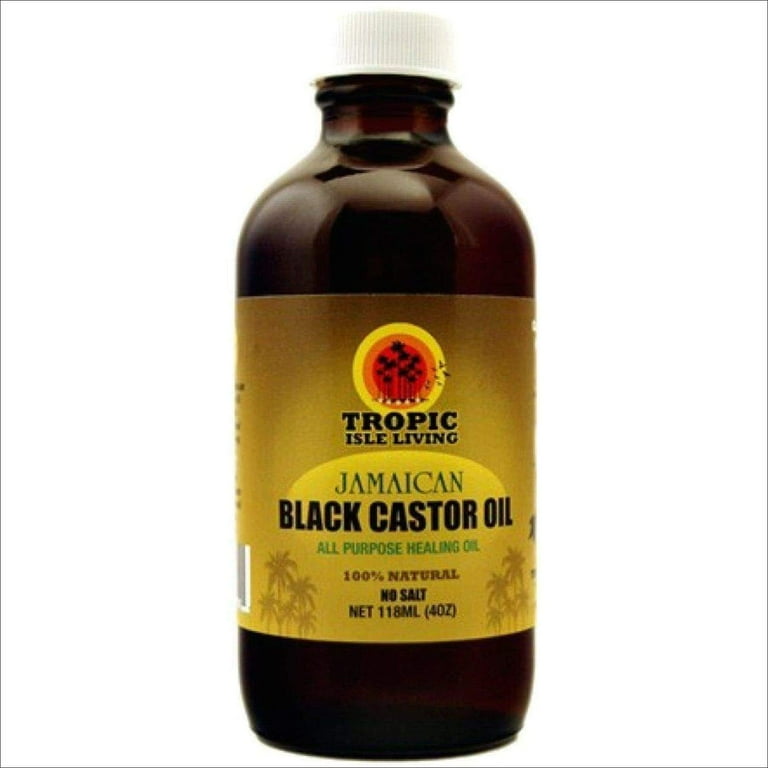The image depicts a brown bottle, likely made of glass or plastic, that contains Tropic Isle Living Jamaican Black Castor Oil. The bottle features a white plastic cap and is wrapped with an orangish-yellow label. At the top center of the label is a distinctive sun-like circular logo displaying silhouettes of palm trees, with concentric circles in yellow, orange, and red hues. Directly below the logo, in bold black letters, it says "Tropic Isle Living." The product's name is clearly stated below in dark green and black lettering: "Jamaican Black Castor Oil," with the phrase "All-Purpose Healing Oil" in green. Further down, it mentions "100% Natural" in brown lettering and "No Salt" in black. The net weight is specified as 118 ML (or 4 ounces) at the bottom of the label. On the left side of the bottle, a UPC code can be seen. The label, although functional, appears somewhat muted and lacks vibrant colors typically associated with health-related products.